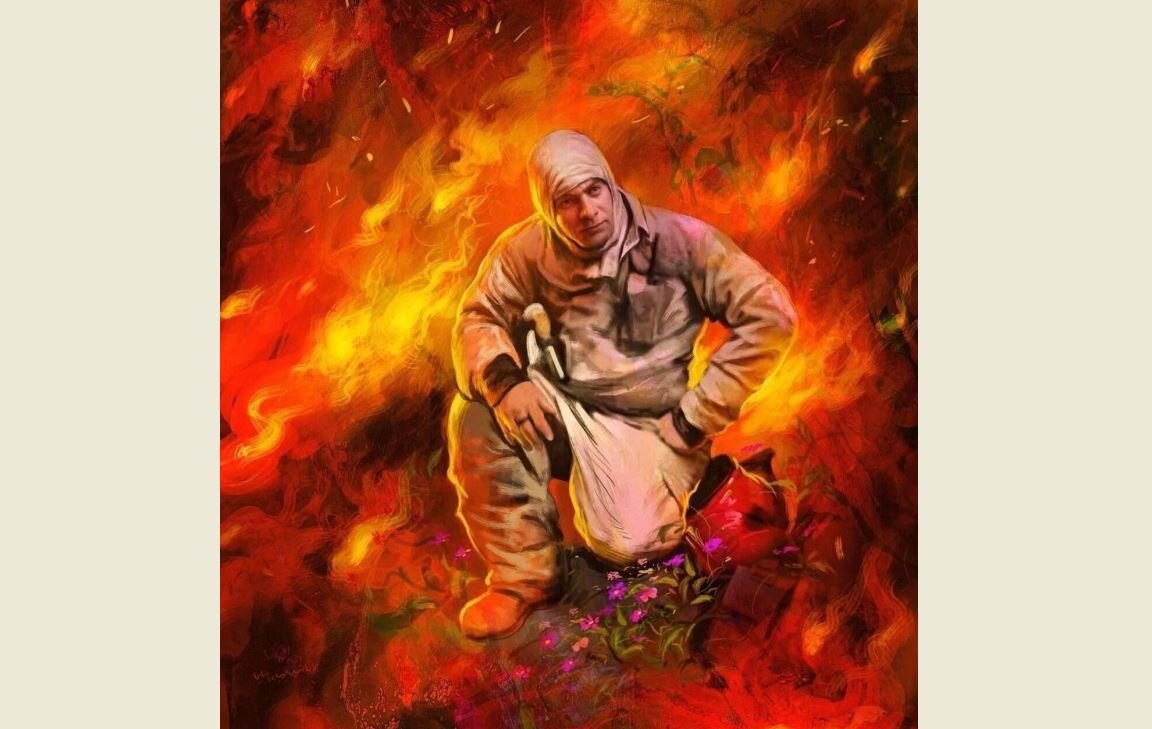In this striking and surreal image, a man is depicted kneeling solemnly before a cluster of delicate pink and purple flowers, juxtaposed against a dramatic, fiery backdrop. He wears a white, protective suit resembling a hazmat outfit, complete with a hood that reveals his entire face. His right arm rests purposefully on his propped-up knee, adorned with a ring on his middle finger, while his left hand is placed confidently on his hip. The scorching flames in the background, painted in vivid oranges and reds, almost seem to reflect off the left side of his clothing, yet don't seem to affect him. The man, equipped with what appears to be tools—possibly a radio or walkie-talkie—tucked into his thick, off-white pants and hinted at a concealed weapon, gazes off to his left with an air of determination. Despite the inferno surrounding him, he appears strikingly composed and unaffected, creating a powerful contrast between the serene foreground and the chaotic, fiery backdrop.